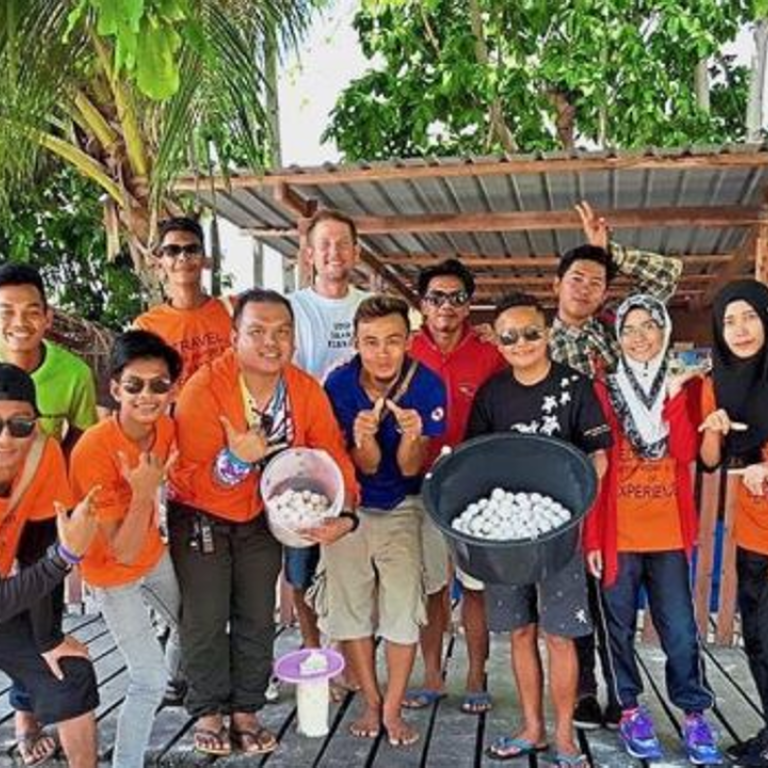This photograph captures a joyful group of twelve predominantly Asian individuals, likely of Filipino or Polynesian descent, gathered outdoors in front of a rustic open shed-like structure. The backdrop features towering tropical trees, including palms and large green leaves, under the clear daylight. The group is dressed in a variety of casual attire, with a notable abundance of orange shirts, hoodies, and aprons, indicating a possible group event or travel-related activity. 

The two women on the right are distinguished by their headscarves; one wears an orange apron over blue jeans and purple sneakers with a black and white head covering, while the other sports an orange shirt, black pants, and a black headscarf. Among the men, diverse clothing includes a plaid shirt, a lime green shirt, and several orange tops. Notably, the Caucasian man in the group stands out with his white t-shirt and blond hair, positioned in the back row.

Two men in the front hold containers filled with white round objects resembling golf balls. One of these individuals wears a black t-shirt with white stars and flip-flops, while the other has on an orange jacket. Many of the group members display hand signs with their thumbs and pinkies extended, adding to the lively atmosphere. The ground they stand on appears to be a wooden porch, with several members in flip-flops or barefoot, and only a few in sneakers. The scene is completed with the group organized in two rows, all beaming at the camera, embodying a sense of unity and celebration.